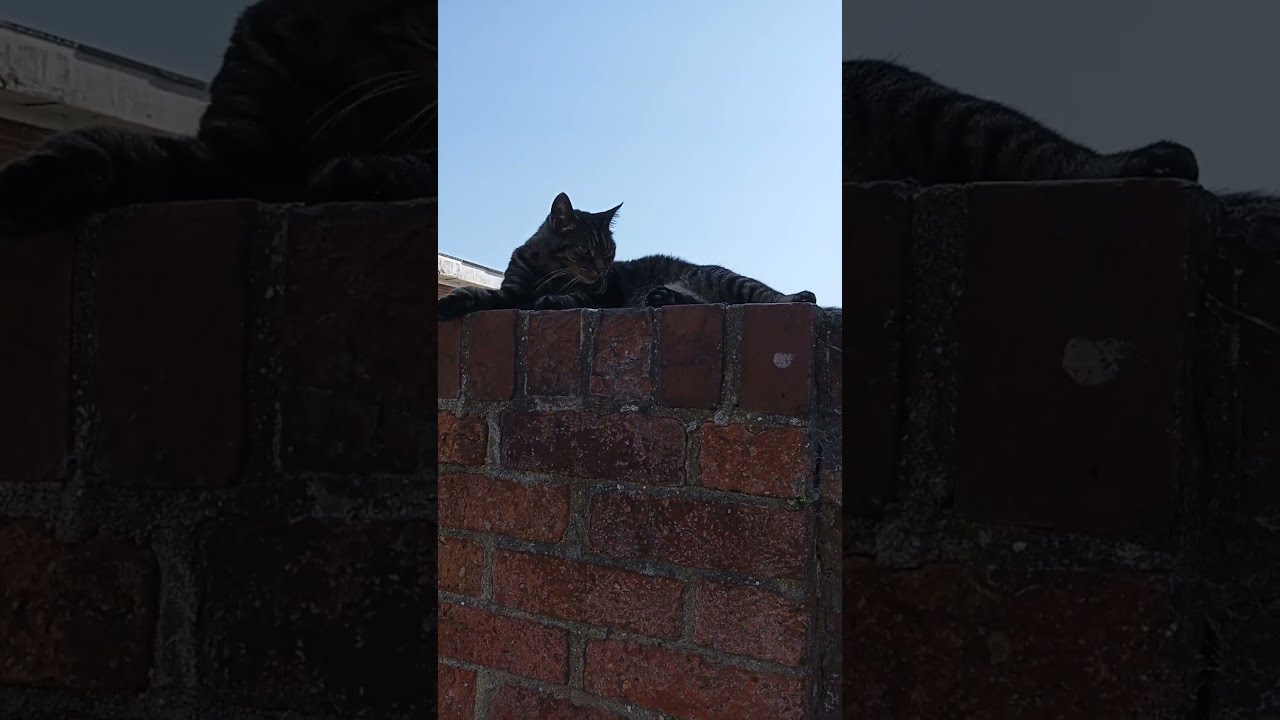In the center of a triptych-style image, a dark gray cat with black stripes lounges on top of a well-weathered red brick wall. The cat, positioned slightly to the left and gazing off to the right, sports long white whiskers and alert ears. The background of the central photo features a bright blue sky with a faint touch of white in the top right corner, hinting at a barely visible cloud. The brick wall, composed of rectangular red bricks, has visible signs of wear with white marks scattered across its surface. The wall’s top is lined with square red bricks. Flanking the central picture are two zoomed-in images; the left one captures the cat's lower half, tail, a portion of the roof, and the top section of the wall, while the right one focuses on the cat’s back, stomach, and back leg against the upper portion of the wall. Both side images are darker, highlighting these specific details.